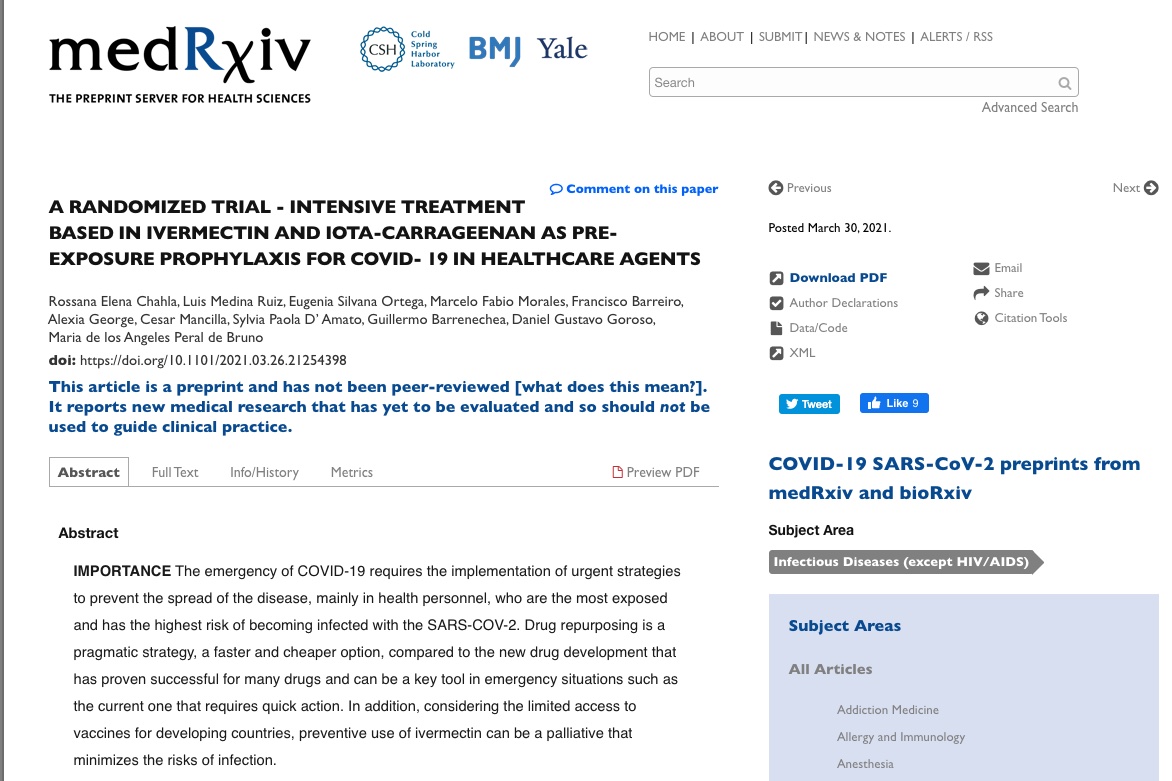**Screenshot of a Medical Journal Abstract**

The image features a screenshot with a white background, showcasing an abstract of a scientific study published in a medical journal. In the upper left corner, the name of the organization, MedRxiv, is displayed. The logo is styled with lowercase black letters spelling "med," followed by an uppercase blue "R," and then lowercase "xiv." Beneath this logo, the phrase "the preprint server for health sciences" is written.

To the right of the MedRxiv logo, several other logos are lined up. The first is the Cold Spring Harbor Laboratory, represented by a circular logo containing the letters "C-H-S." Next to it is "BMJ" for the British Medical Journal, displayed in capital letters. Following this, in light gray letters, is "Yale."

Across the top right, a menu is written in light gray capital letters, listing options such as "HOME," "ABOUT," "SUBMIT," "NEWS & NOTES," "ALERTS," and "RSS." Below this menu is a long rectangular search box.

On the left side of the image, the title of the research paper is prominently displayed in bold black font: "A Randomized Trial: Intensive Treatment Based on Ivermectin and Iota-Carrageenan as Pre-Exposure Prophylaxis for COVID-19 in Healthcare Agents." Directly beneath the title, the authors' names are listed in a smaller, gray font.

Further down, in bold blue font, a disclaimer states, "This article is a preprint and has not been peer-reviewed." In brackets, it prompts the reader with "[What does this mean?]" A subsequent note elaborates that the article reports new medical research that has yet to be evaluated, and therefore, should not be used to guide clinical practice.

Finally, the abstract itself is presented, summarizing the study's aim to investigate the efficacy of intensive treatment incorporating ivermectin and iota-carrageenan as pre-exposure prophylactic measures against COVID-19 in healthcare settings.